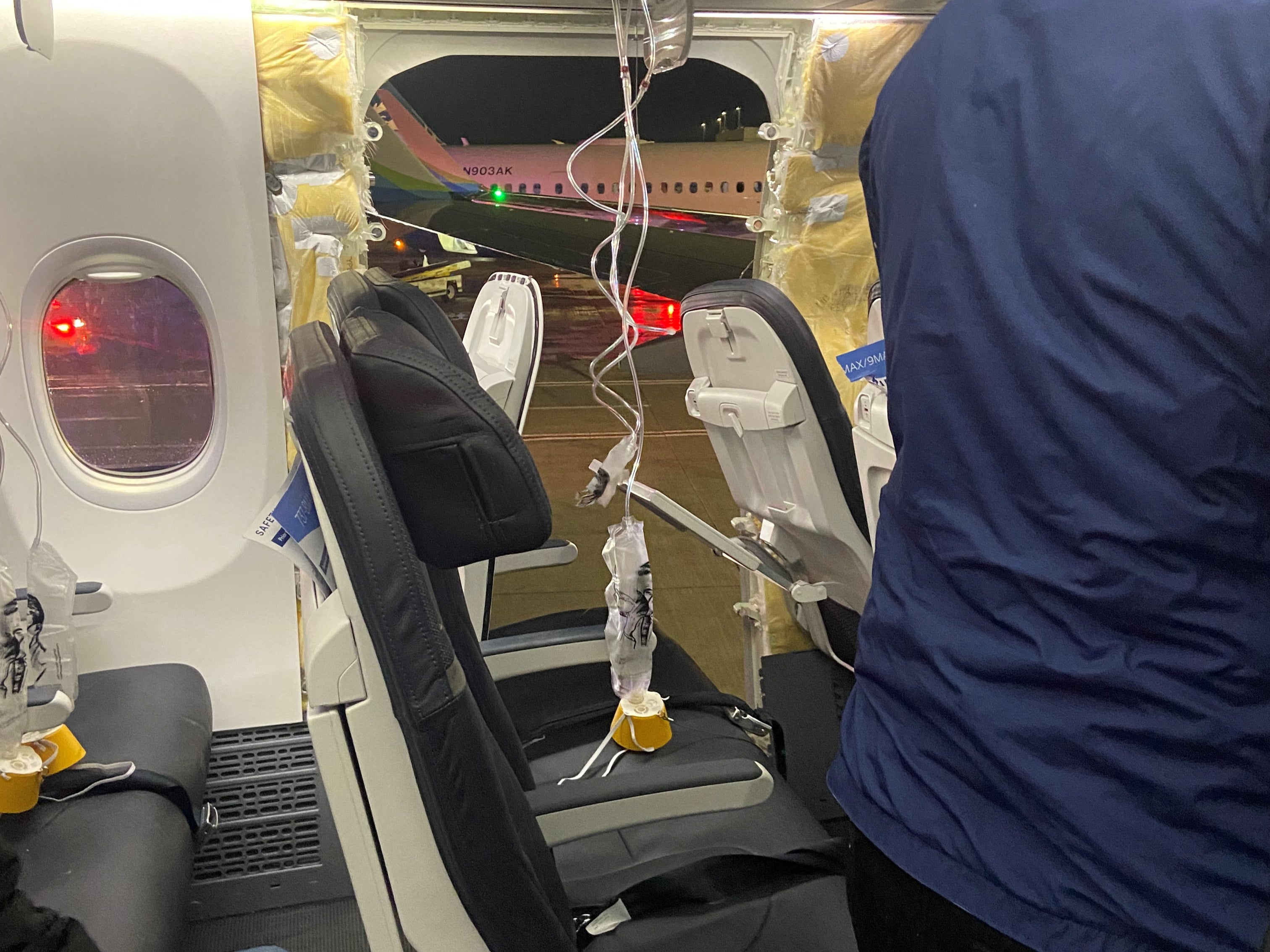The image captures a tense scene inside the cabin of an airplane that appears to have made an emergency landing. The photo is taken from within the plane, with a clear view of a gaping hole near a row of black seats, which looks to have resulted from decompression. Through this opening, the night sky and a distant, stationary airplane on the tarmac can be seen, confirming the plane has landed.

Inside the cabin, the aftermath of the emergency is evident. Oxygen masks and the clear plastic tubes designed to deliver oxygen in case of cabin pressure loss are hanging down from the overhead compartments, draping onto the seats. The interior panels around the emergency door are frayed and damaged, indicating a violent incident. The red emergency lights are casting a dim glow across the chaotic scene.

In the foreground, the back of a man wearing a dark blue shirt and black pants is visible. His pose suggests he's looking towards the aftermath of the decompression event, adding a human element to the scene. The overall atmosphere is one of intense disorder and relief, showing the plane's interior after what was likely a harrowing emergency landing.